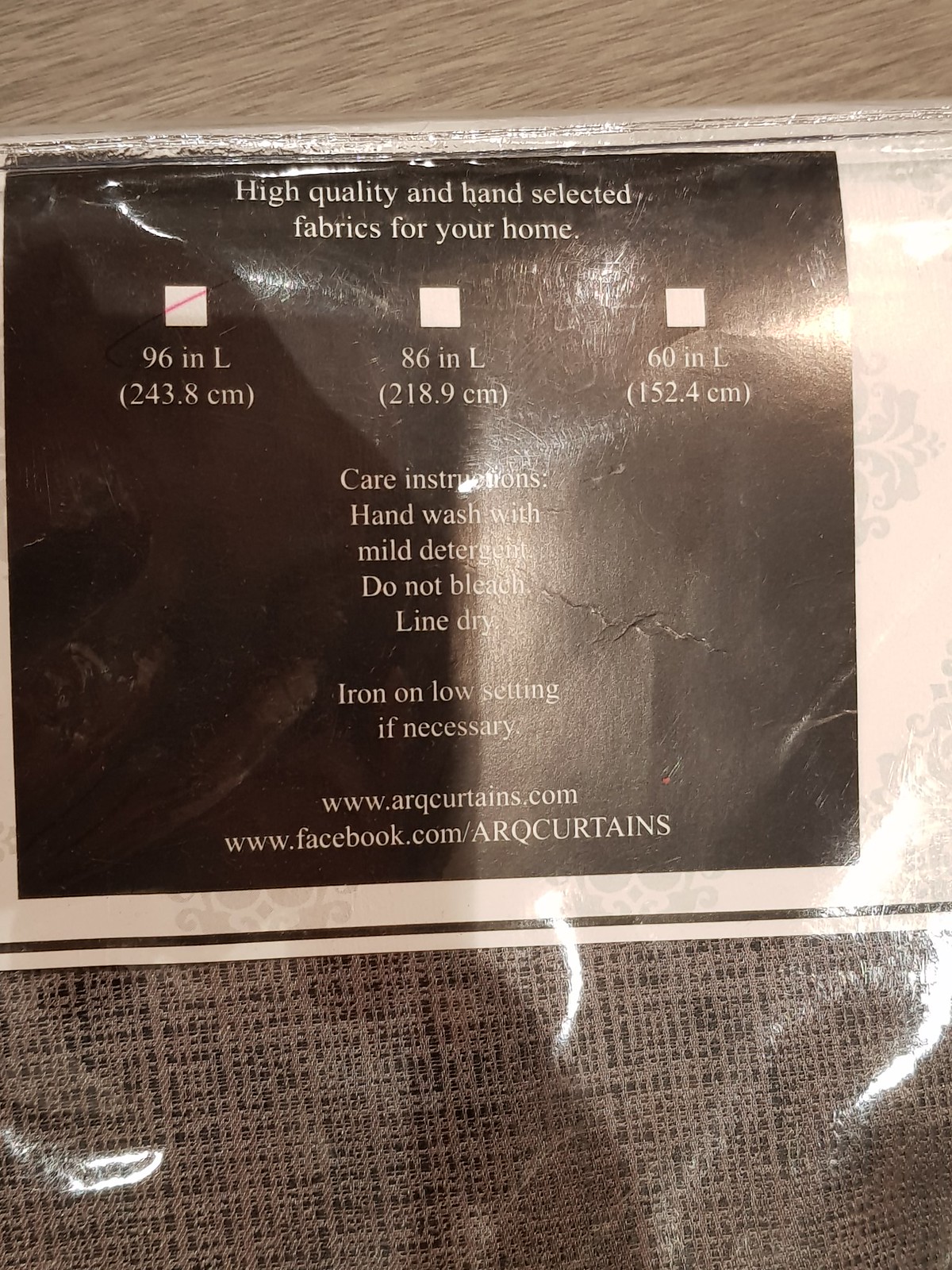Here is the detail-oriented and cleaned-up caption for the image:

---

The image showcases the back of a pack of curtains. The curtains appear to have a brown and black thatch pattern. The packaging highlights that the curtains are made from high-quality, hand-selected fabrics ideal for home decor. They are available in three sizes: 96 inches, 86 inches, and 60 inches. The specific pack in the image contains curtains that are 96 inches in length.

Care instructions provided on the package are as follows:
- Hand wash with mild detergent
- Do not bleach
- Line dry
- Iron on a low setting if necessary 

For more information or to purchase, you can visit their website at www.arqcurtains.com or their Facebook page at www.facebook.com/ARQcurtains.

---